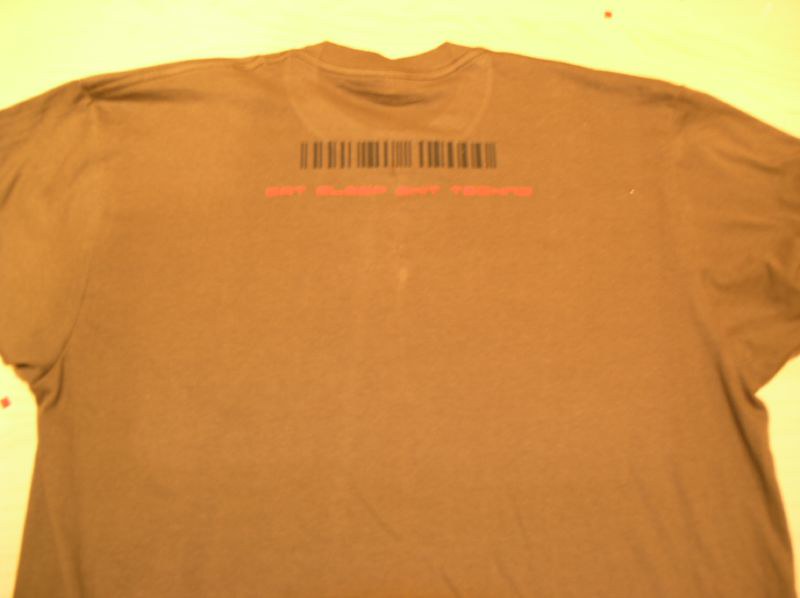This is a close-up color photograph of a worn orange short-sleeve crew cut t-shirt laid flat on a yellow surface. The image is slightly wider than it is tall and is cropped mid-waist and just past the armpits of the shirt. At the top front of the t-shirt near the neck, there is a black barcode with bright orange or pink writing underneath it, which appears wavy and indicates that it has been worn. The text is not legible. The rest of the t-shirt is plain and shows some wrinkles. The photograph was taken from the bottom of the t-shirt looking up towards the neckline. There are no other objects, people, animals, plants, buildings, signs, or vehicles in the image.